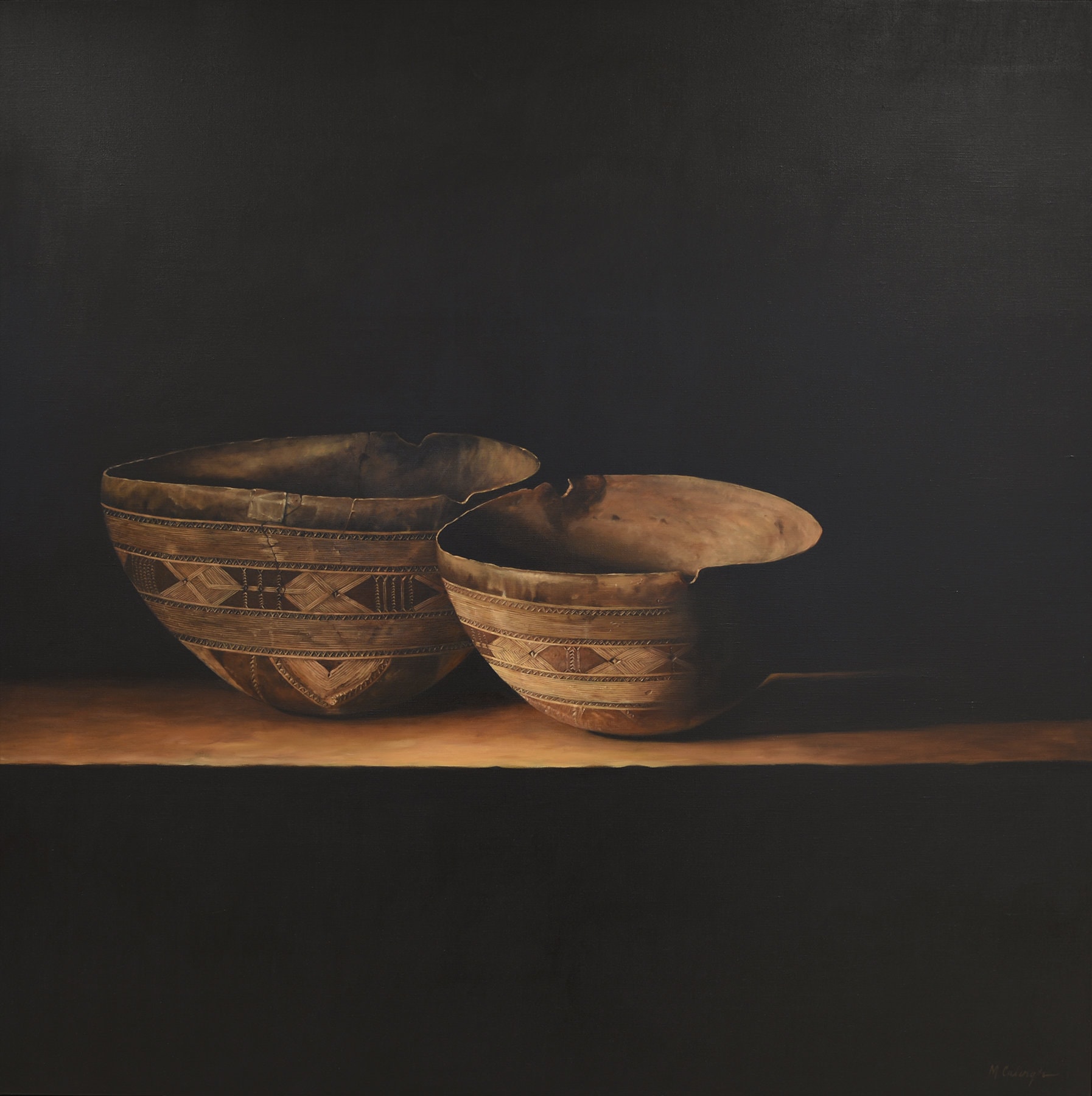This image features two antique, weathered bowls placed on a light brown wooden shelf within a predominantly dark environment. It appears to be an illustration, possibly an oil painting, depicting the bowls with considerable attention to their historical and artistic elements. The bowls, which might be crafted from clay or ceramic (possibly even wood with designs carved onto them), exhibit a range of earthy tones, from beige and dark brown to reddish hues. Both bowls display consistent chipping along their rims, suggesting either age or a decorative intent.

Each bowl is adorned with intricate, multi-colored geometric patterns, including triangles and circular designs evocative of ancient Native American or Aztec artistry. The bowl on the right is smaller, while the one on the left is larger. The shelf itself is illuminated, highlighting the detailed designs on the bowls, while the backdrop remains pitch black, drawing focus entirely to these historical artifacts.